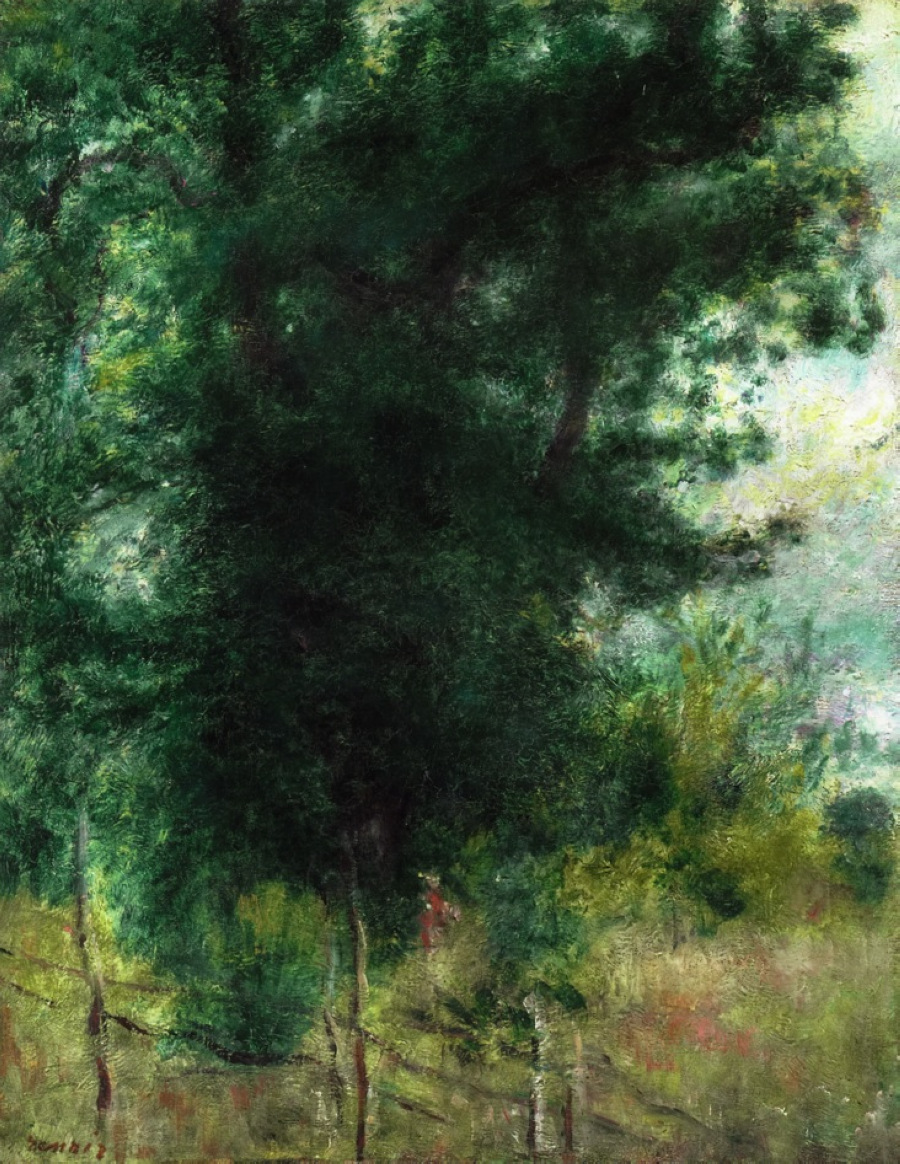This image captures a Monet-style painting characterized by its use of small, colorful brushstrokes forming a cohesive scene. The painting is in portrait orientation, dominated by a towering, dark green tree centrally positioned. At the bottom left, a detailed, rickety wooden fence painted in shades of brown stretches towards the bottom center. Surrounding the main tree are other trees in lighter green tones, creating depth in the background.

The ground consists of grass in a variety of green and gold shades, leading up to the fence. Just above the fence, slightly towards the left, there's a subtle depiction of a person in a red dress with light skin. On the right side of the painting, through the tree branches, hints of light blue sky are visible. The artist's signature, although present in the bottom left corner, remains unreadable due to its small size and blending with the background. The painting's assembly of colors, including brown, green, gold, red, yellow, and blue, evokes a vibrant outdoor scene that could be showcased in a museum or art show.